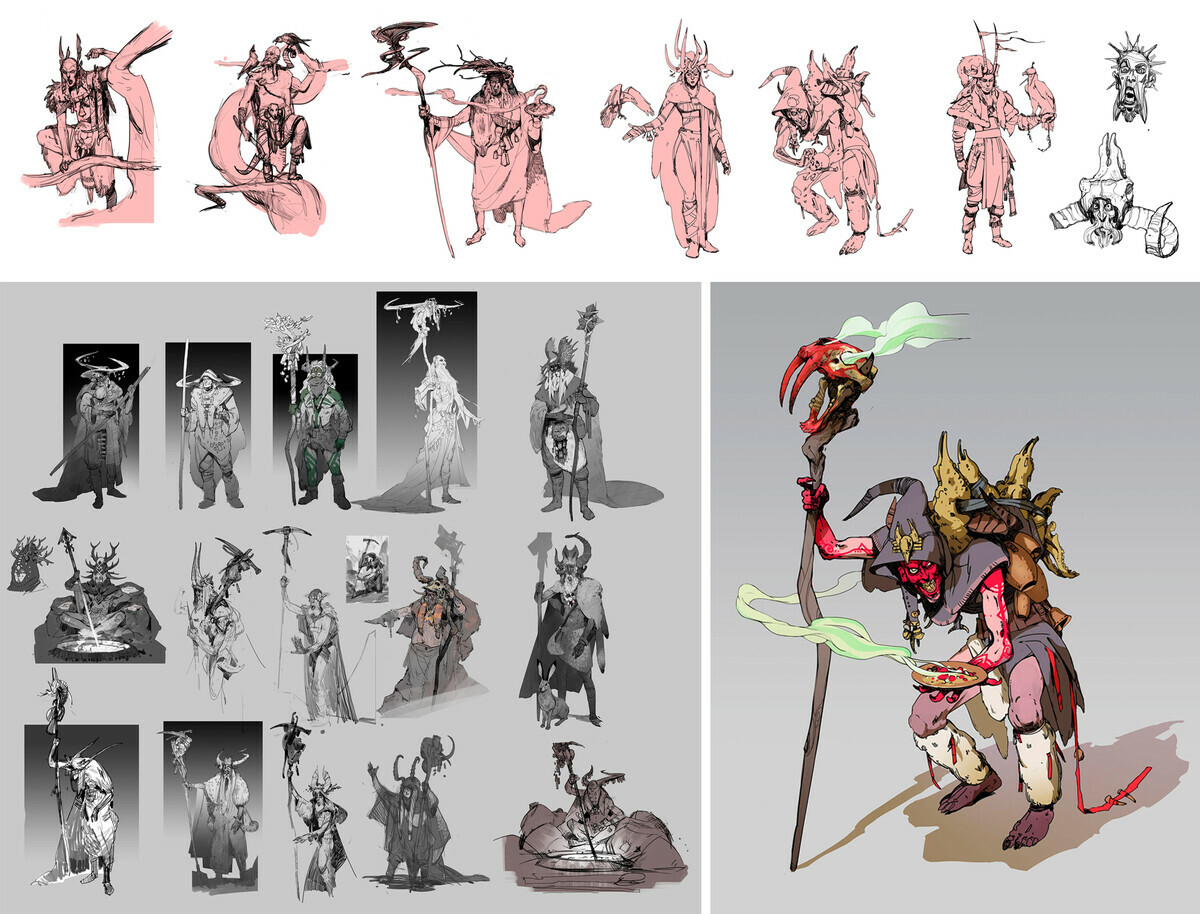The image showcases a striking triptych of concept art for fantasy characters, displaying a consistent, eerie theme. At the top, there are six pink-colored, shadowy figures of various monstrous beings, the final one being a simple hand drawing of a head. Beneath this, on the left side, is a gray-toned section with columns of smaller, indistinct figures arranged in a grid of five across and three down. These appear to be characters from a game or a fantastical future setting, though the details are too minute to discern clearly. Finally, occupying the bottom right, is a more detailed depiction of a singular, vividly colored character. This shamanic figure, combining elements of both the pink figures and the black and white tones, has a menacing red devil face and wears a gray cloak. The character, adorned with tribal accoutrements like horns and animal furs, clutches a staff topped with a skull featuring long red fangs and has a dish emitting smoke. He crouches, revealing monstrous feet with claws and carries an additional object on his back. The palette predominantly features pinks, blacks, whites, and splashes of red, enhancing the eerie, tribal aesthetic.